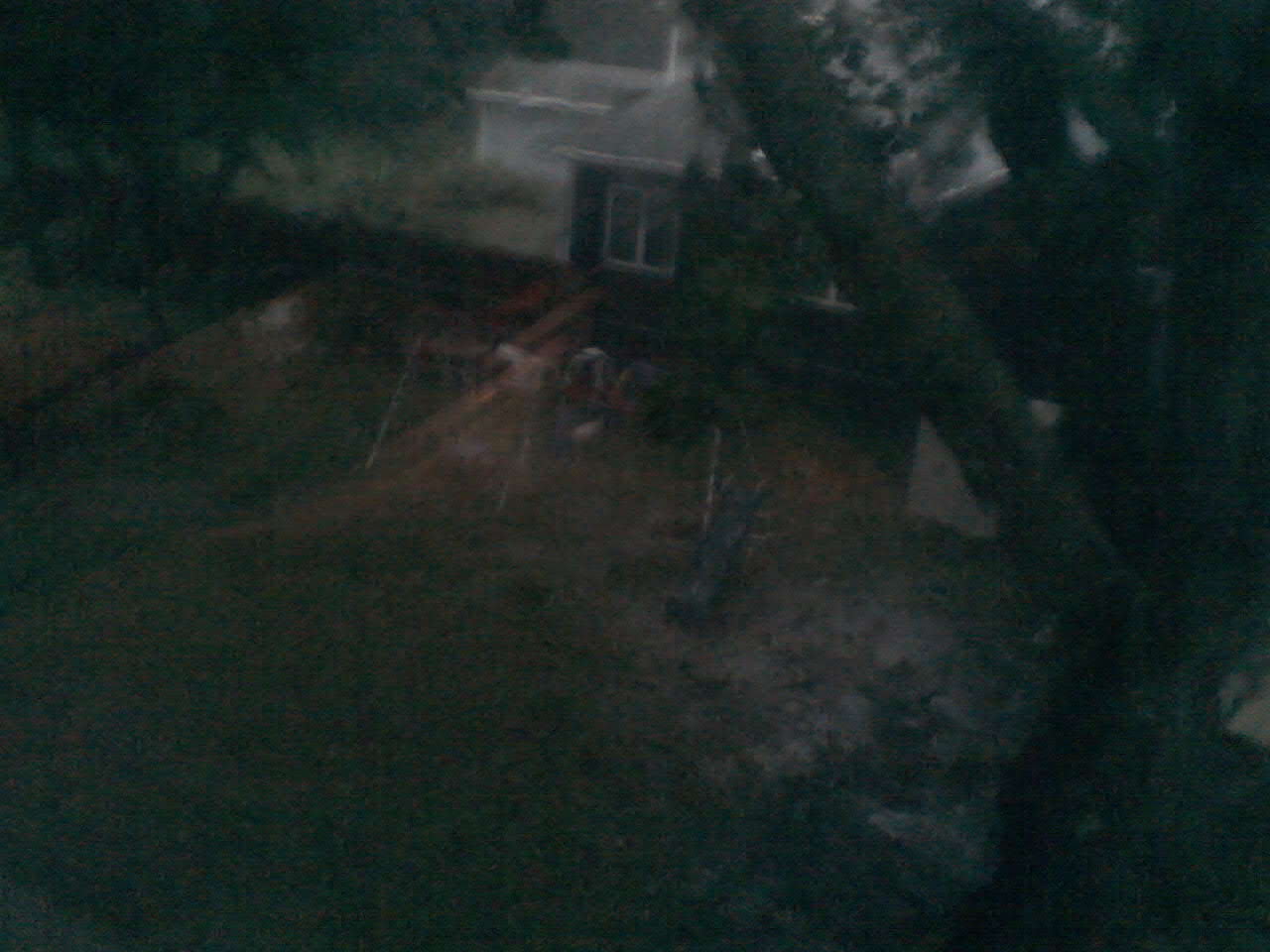The photograph is a blurry, dark image of a backyard taken either in the evening or under low-light conditions, making it hard to discern many details. However, the green grassy yard is visible, along with a large tree with green leaves. The backyard features a swing set with a dark green plastic slide, and scattered toys that suggest it might be a child's play area. There are also indications of a clothesline in the yard. The house at the back has dark-colored walls and a grey roof with white guttering. The windows have white frames, and beside the house, there is a small white garage or outbuilding. The image's poor focus and low light make it difficult to tell more specific details about the materials or additional features.